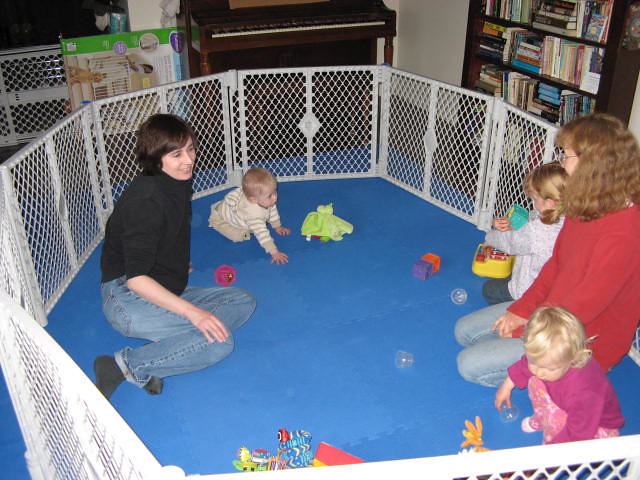The photograph captures a lively daycare setting where a white playpen, marked with a mesh design and placed over a large blue mat, encloses three children—one baby, one toddler, and an older toddler—all engaged with various colorful toys. Prominent toys include square blocks and a toy xylophone, alongside vibrant pink, orange, blue, and red toys scattered on the playpen's floor. Two women, presumably caregivers, are within the playpen monitoring and interacting with the children. The woman on the left, wearing a black sweater, blue jeans, and black boots, is lying on her side, while the woman on the right, donned in a red sweater and blue jeans, kneels attentively. The child in the bottom left corner is dressed in a pink jersey and trousers adorned with designs, while another child on the right side, wearing a grey jersey and blue jeans, holds a blue toy. Beyond the playpen, the room features a brown piano and a cabinet filled with books, adding to the daycare's warm and educational atmosphere.